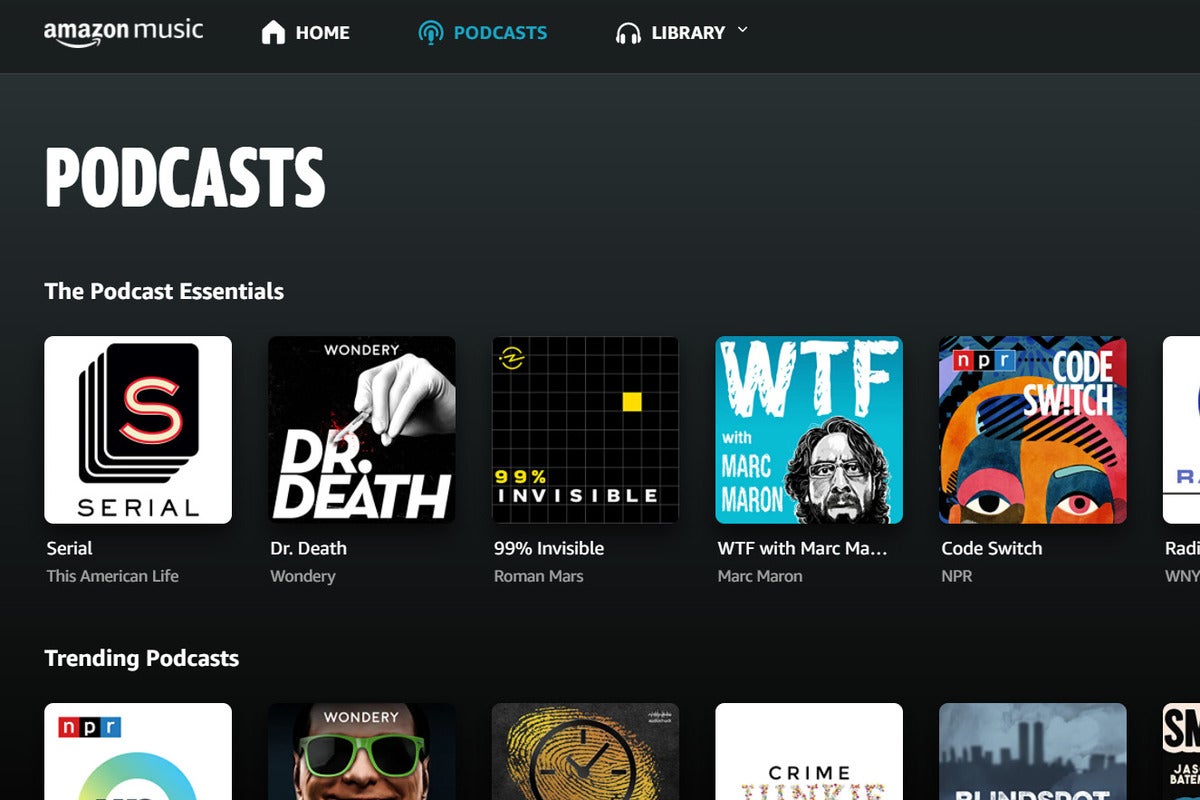The image depicts the podcast page within the Amazon Music application, showcasing a sleek, dark-themed interface. The background transitions from deep black to lighter shades of gray towards the upper left corner. At the top, a solid black header bar spans across the page, displaying the Amazon Music logo featuring the iconic Amazon arrow connecting the "A" and "Z" beneath the brand name.

Three selectable tabs are present within this header: Home, Podcasts, and Library, each accompanied by a corresponding icon — a house for Home, an exclamation mark with emanating semi-circles for Podcasts, and over-the-ear headphones for Library. The Podcasts tab is highlighted in a teal blue, indicating it is currently selected, while the Home and Library tabs appear in white.

In the upper left section of the main page, bold, all-caps text reads "PODCASTS," followed by "Podcast Essentials" beneath it. Below this heading is a row featuring five distinct podcast thumbnails with rounded corners, each representing different shows: 

1. **Serial** by This American Life - Depicted as an "S" with an orange outline resembling a stack of four books.
2. **Dr. Death** by Wondery - Showcasing a striking image relevant to the podcast.
3. **99% Invisible** by Roman Mars - Featuring its signature design motif.
4. **WTF with Marc Maron** - Displayed as "WTF with MarkMA..." reflecting a partial view of the title.
5. **Code Switch** by NPR - Shown with a neatly designed thumbnail.

A hint of a sixth podcast, likely "Radiolab" by WNYC, is partially visible on the far right, with the remaining part cut off.

Below this row lies another partially obscured row labeled "Trending Podcasts," displaying several podcast thumbnails. Among them are recognizable designs from NPR and Wondery, along with a fingerprint and a clock, a cityscape, and a thumbnail with the text "True Something." Another thumbnail shows partial text "S..." possibly followed by "N" or "M," and the partial author name "JASBAT," further cut-off.

Overall, the page offers a visually rich and intuitive podcast browsing experience within the Amazon Music app.